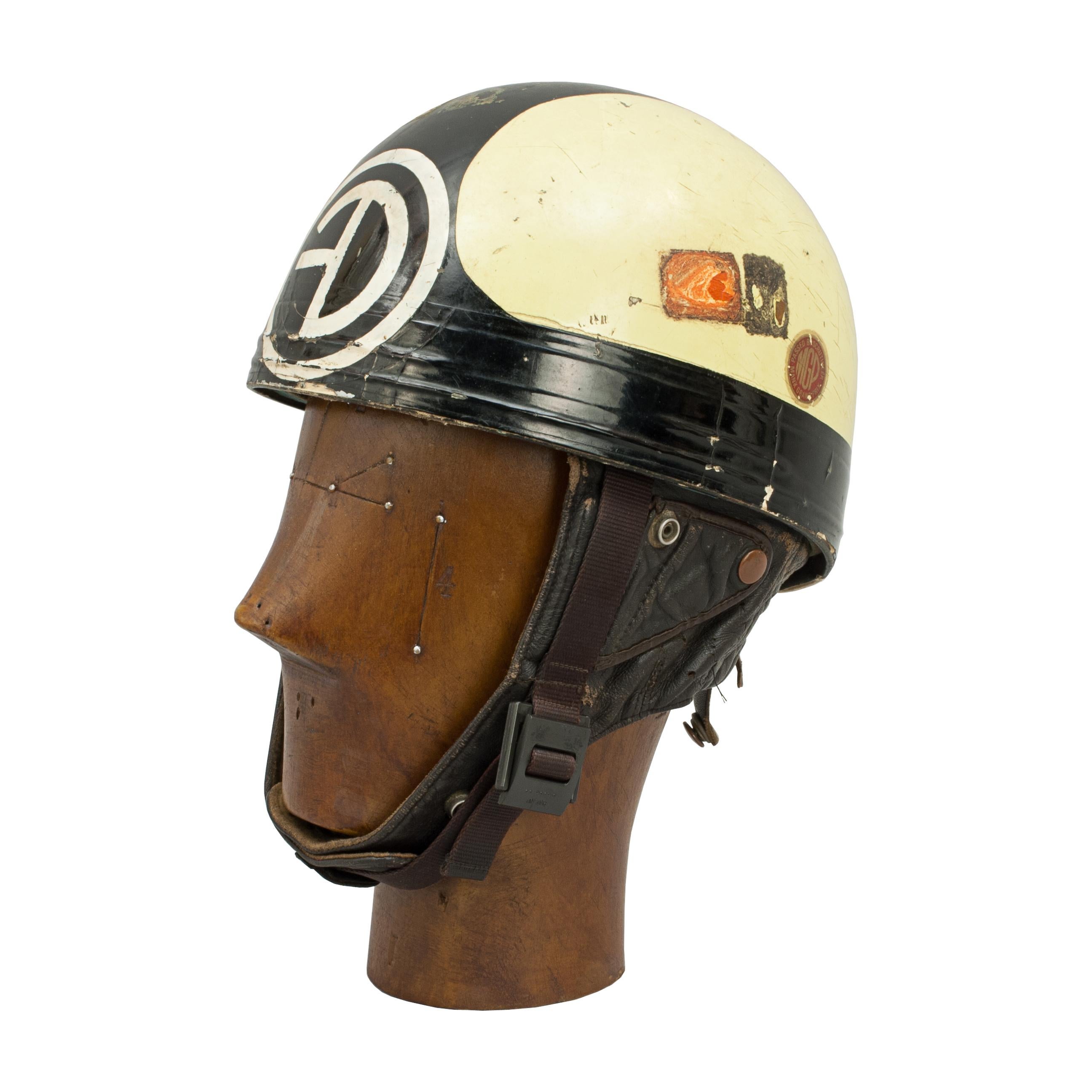The image depicts a dark wooden mannequin head, likely from an antique shop or a selling platform, characterized by minimal facial features with pin markings indicating facial points such as the cheek area and eye positions, and a prominent wooden nose. The mannequin is adorned with a worn helmet, distinguished by its black and cream coloration. The helmet features a central black stripe, a white circle on the front with lettering that appears to form "DF", and several faded, dirty stickers on the white sections near the sides, which look like old postage stamps. Additionally, the helmet has a fabric covering over the ears and a vinyl and leather strap extending from the sides of the face down to underneath the chin. The background of the image is entirely white, ensuring full focus on the detailed presentation of the mannequin and helmet, adding a historical or vintage feel reminiscent of old policeman's headgear.